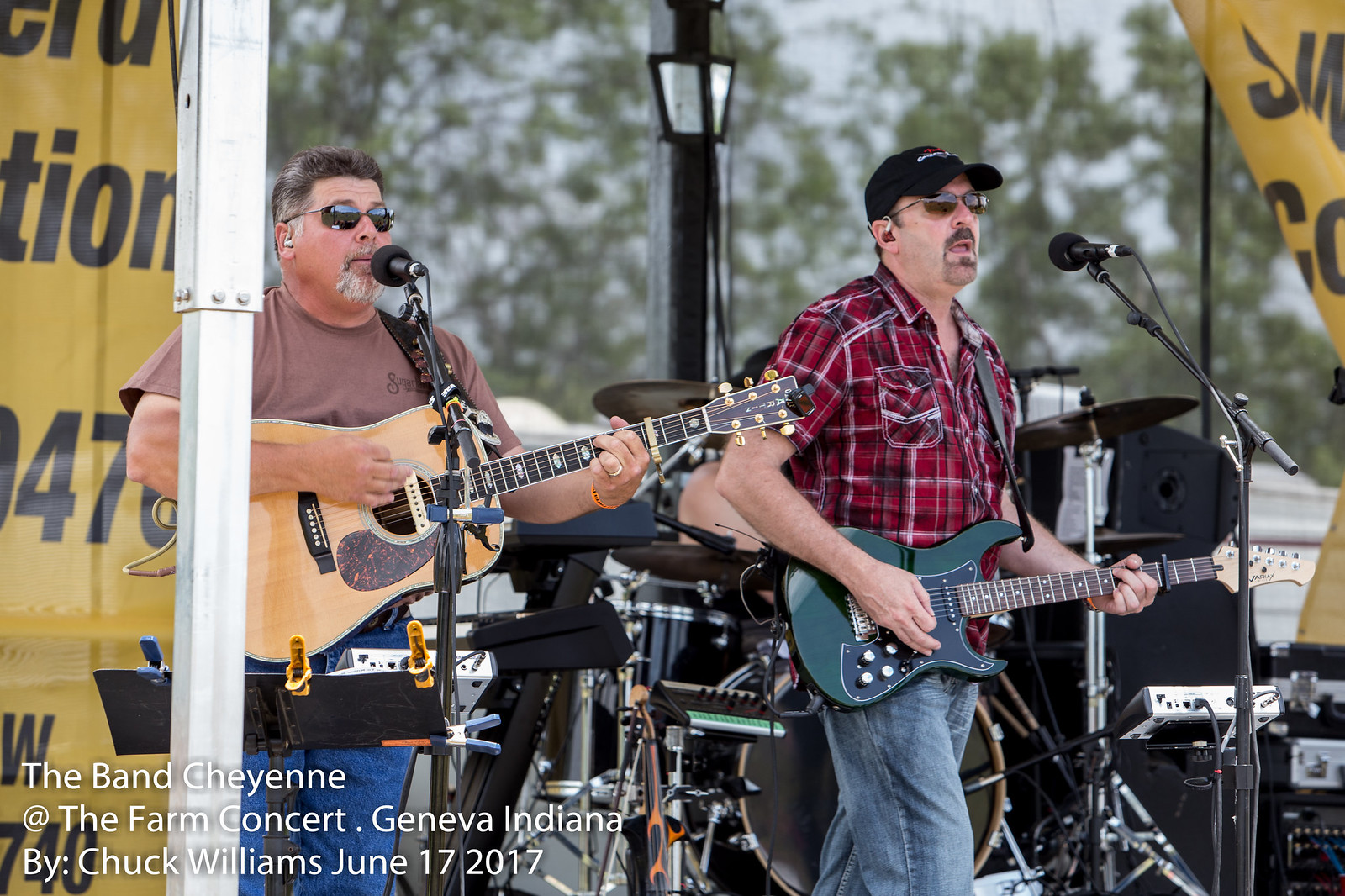This detailed photograph captures a live outdoor performance by the band Cayenne at the Farm Concert in Geneva, Indiana, on June 17, 2017, credited to Chuck Williams. The scene is set under a tent with lights mounted on poles, indicating a bright, sunny day with blurred trees in the background. The focus is tight, primarily showcasing two musicians on stage mid-performance, both singing into microphones on stands.

On the right, a musician clad in a white, black, and red checkered flannel shirt, blue Levi jeans, sunglasses, and a black baseball cap with a logo stands playing a green electric guitar with a black pick guard. He also has ear monitors. To his left, another musician sports a brown t-shirt, blue Levi jeans, sunglasses, and a goatee, strumming a light maple wood-colored acoustic guitar. Both are engaged with their microphones, delivering vocals.

Partially visible in the background is a drum set, though the drummer remains obscured due to the tight framing and positioning of the guitarists. The lower left corner of the photograph features medium white text stating, "The band Cayenne at Farm Concert, Geneva, Indiana by Chuck Williams, June 17, 2017."